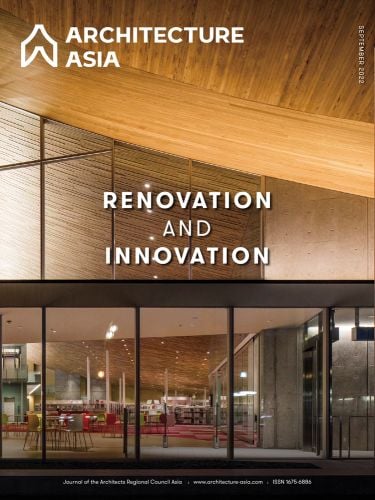This advertisement for the architectural store "Architecture Asia" is a detailed photograph showcasing the interior of a modern architectural showroom. The image features a slanted wooden ceiling with both light and dark brown hues. The store's large glass windows provide a clear view inside where various furniture sets—tables, chairs, and shelving—are displayed, emphasizing the theme of renovation and innovation. At the top of the image, the store's name "Architecture Asia" is prominently displayed in white text, accompanied by a distinct logo resembling an upside-down Y shape. Centered in the photograph is the phrase "Renovation and Innovation," also in white text. The bottom part of the advertisement contains a black border with small white text, providing contact information such as the Journal of Architects details, a website, and a phone number, though the text is difficult to read.